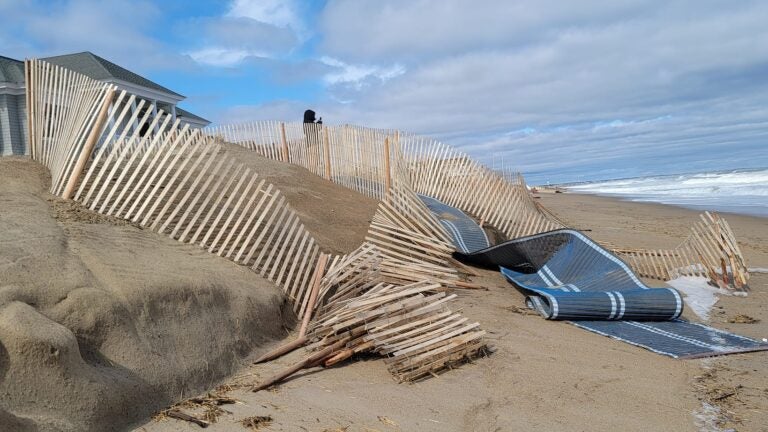The image depicts a beach scene, possibly an artistic rendering. The beach is characterized by a sandy stretch and a smooth rock toward the left-hand side. A prominently fallen wooden fence, likely a snow fence, winds through the scene in disarray, stretching from the beach to a sandy hill that leads up to a house with a gray roof, partially obscured by the fence. The fence is beige and appears to have been knocked down, spreading across the sand alongside a crumpled and partially blown-away blue mat with white stripes. The sky above showcases a mix of bright blue on the left, gradually blending into horizontal layers of gray and white striated clouds to the right. This cloudy expanse makes it difficult to distinguish where the sky ends and the dark blue ocean, frothing with white foam at the edges, begins. In the background, a silhouette of a woman, possibly capturing a photograph, adds a human touch to the tranquil yet slightly disorderly beach scene. Large boulders are scattered behind the fence, contributing to the rugged landscape.